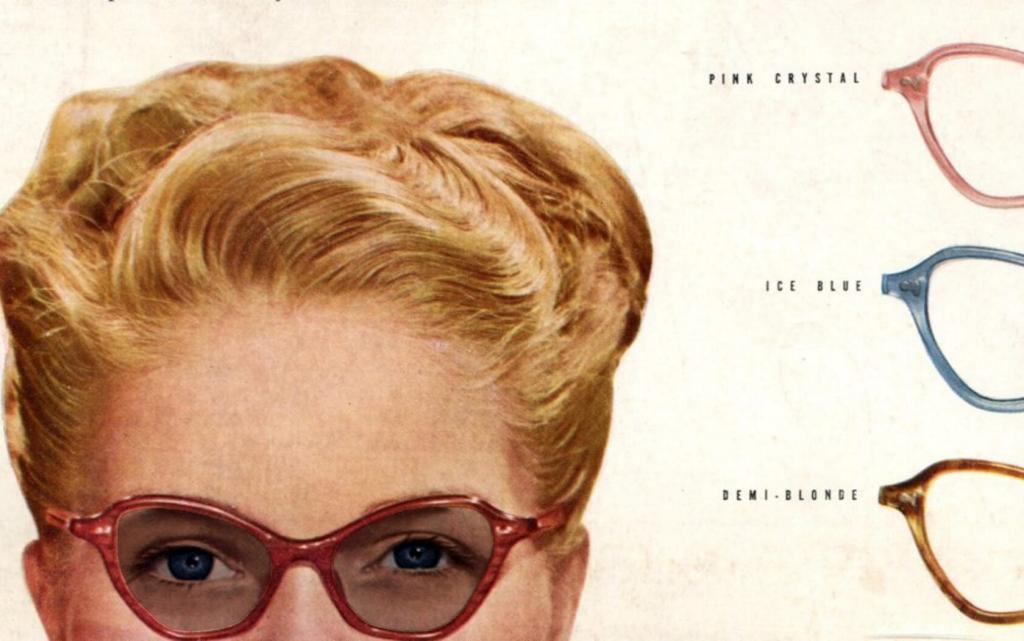In this horizontal image resembling a vintage advertisement, the upper half of a woman's face is prominently featured. She has short, dirty blonde hair combed back and is wearing red-rimmed eyeglasses with slightly tinted lenses, allowing a view of her blue eyes. The woman appears to be modeling the eyeglass frames. The background is entirely white, keeping the focus on the subject and the eyeglass frames.

To the right of the woman's face, there are three eyeglass frames displayed vertically. These frames, identical in shape but varying in color, are labeled as follows from top to bottom: "Pink Crystal" which is a light pink, "Ice Blue" which is a grayish-blue, and "Demi-Blonde" which features a brown and yellow tortoiseshell pattern. Only a portion of each frame is visible, emphasizing the distinctiveness of their colors and designs.